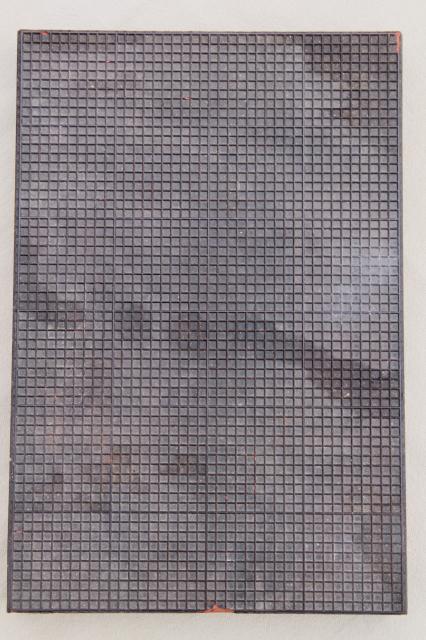This artwork features a slightly tilted, black metal grid screen against a solid gray background. The grid is composed of numerous tiny squares arranged in vertical and horizontal lines, creating an intricate pattern of approximately 50 squares horizontally and 100 vertically. The screen exhibits areas of wear and tear, with varying textures and colors throughout, including dark and brown spots suggestive of dirt. The bottom part of the screen appears particularly damaged, marked by a notable orange segment, possibly indicating rust or breakage. The background lightens in places, resembling clouds, which contrast against the grid. The scene is devoid of any human figures or recognizable images, focusing entirely on the complex interplay of the grid's imperfections and the ethereal background.